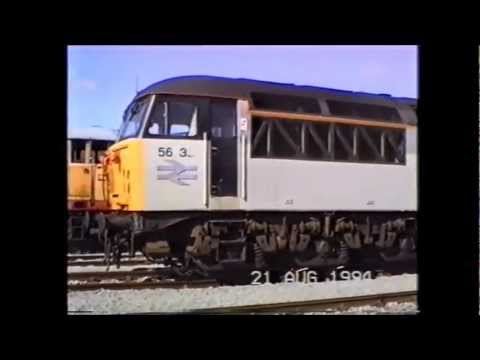This image captures an old photograph of a train with a significant black border framing the entire scene, reminiscent of a still shot from an older home movie, distinguished by a time stamp in the bottom right-hand corner reading "21st August 1994." The photograph prominently features a white train with a yellow-orange front and a black roof. The driver's cab includes a black window with bars and two smaller windows above it; beneath the main window, the number "56.3" is visible. The train's undercarriage, showcasing its wheels and mechanical parts, is black. The tracks beneath the train consist of white gravel and brown rails. In the background, a small portion of another yellow train can be seen, hinting at a more extensive railway system. Overall, the image's composition, combined with the distinct black border, evokes the look and feel of a 1990s-era film still.